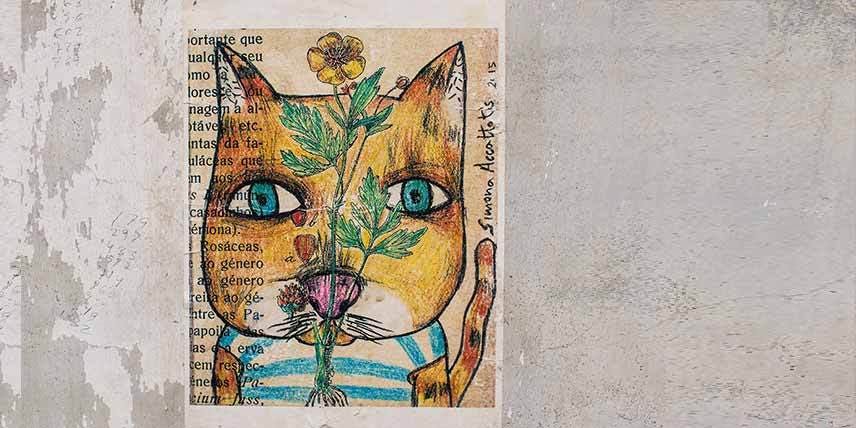In this children's storybook-style illustration, a whimsical anthropomorphic cat with an orange and black tabby pattern and large blue eyes is depicted. The cat, whose body is clothed in a white and blue striped t-shirt, appears cheerful as it holds up a tall yellow flower with green leaves and stems. The drawing, likely created with colored pencils or crayons, features a hand-drawn quality against a contrasting background that resembles a gray, concrete-like surface or abstract black-and-white newsprint. This background frames the central square image of the cat. The top left corner of the illustration includes Spanish text, while the right side prominently displays the artist's name, "Simona Cadantes 2115." The scene is both whimsical and detailed, capturing the playful essence of the cat and the surrounding elements.